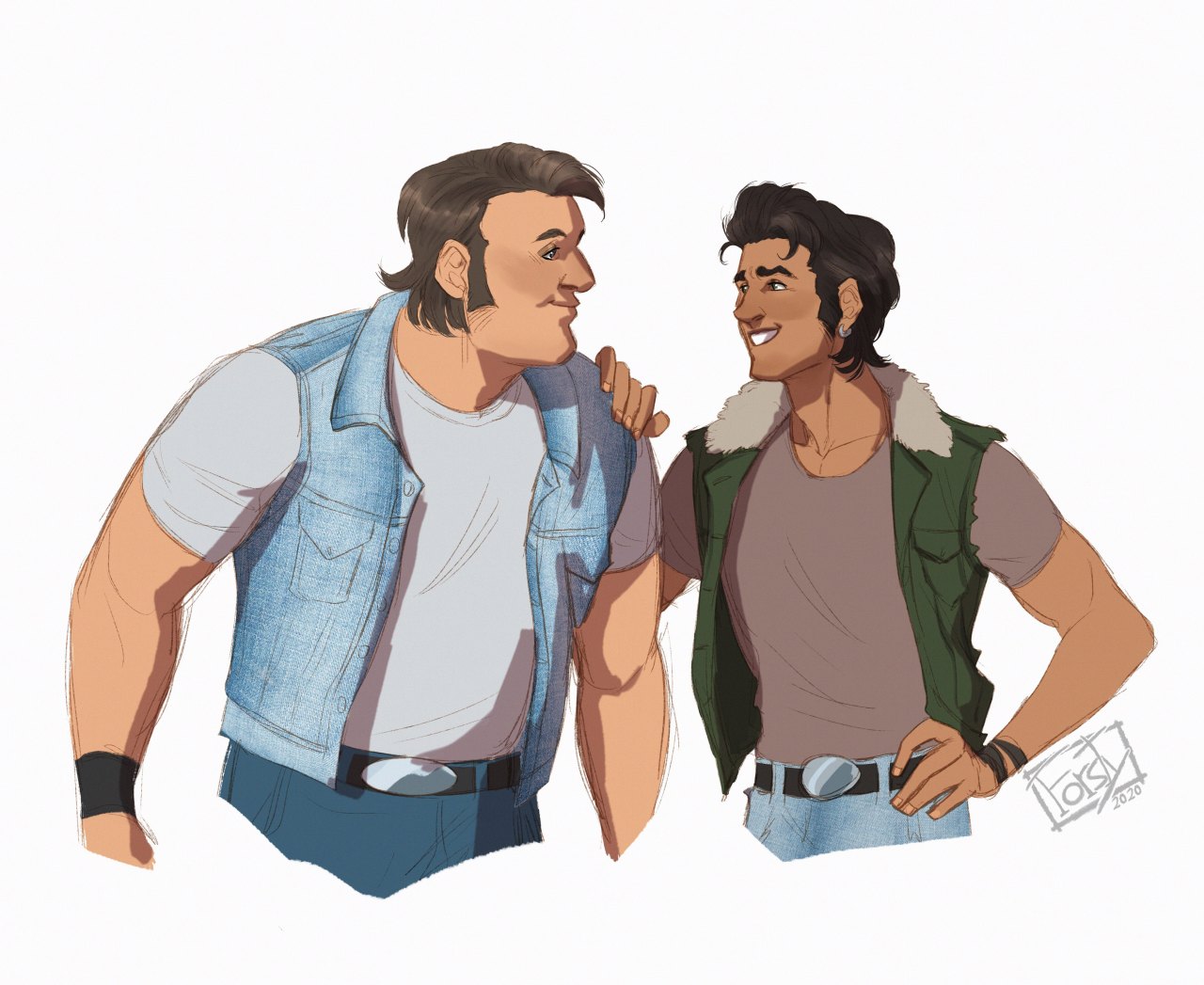The image shows a detailed, possibly computer-generated or painted illustration, reminiscent of a comic book style, against a pure white background. Central to the image are two cartoon-like men depicted from below the belt upwards. 

On the left stands a noticeably bigger, muscular man with broad shoulders and defined biceps. He is clean-shaven and has brown hair with long sideburns, styled in an old-school shaggy cut that falls to below his ears. His attire includes a grey, round-neck, short-sleeved t-shirt, over which he wears a sleeveless denim vest with a collar. He completes his look with blue pants (jeans) and a black belt. Additionally, he sports a black wristband. This character appears to be smiling as he looks at the other man.

The other man, positioned to the right, has a slender yet muscular build. His hair is long and dark, with an earring in one ear, and he appears to be more dusky in complexion. He wears a brown, round-neck, short-sleeved t-shirt, paired with a green sleeveless jacket with fur around the collar. He is also dressed in blue jeans with a black belt and wears bracelets on his left wrist. His right hand is placed on the shoulder of the man on the left, and he seems to be either talking or smiling at him.

At the bottom right corner of the image, there's a watermark that reads "Force Team 2020."